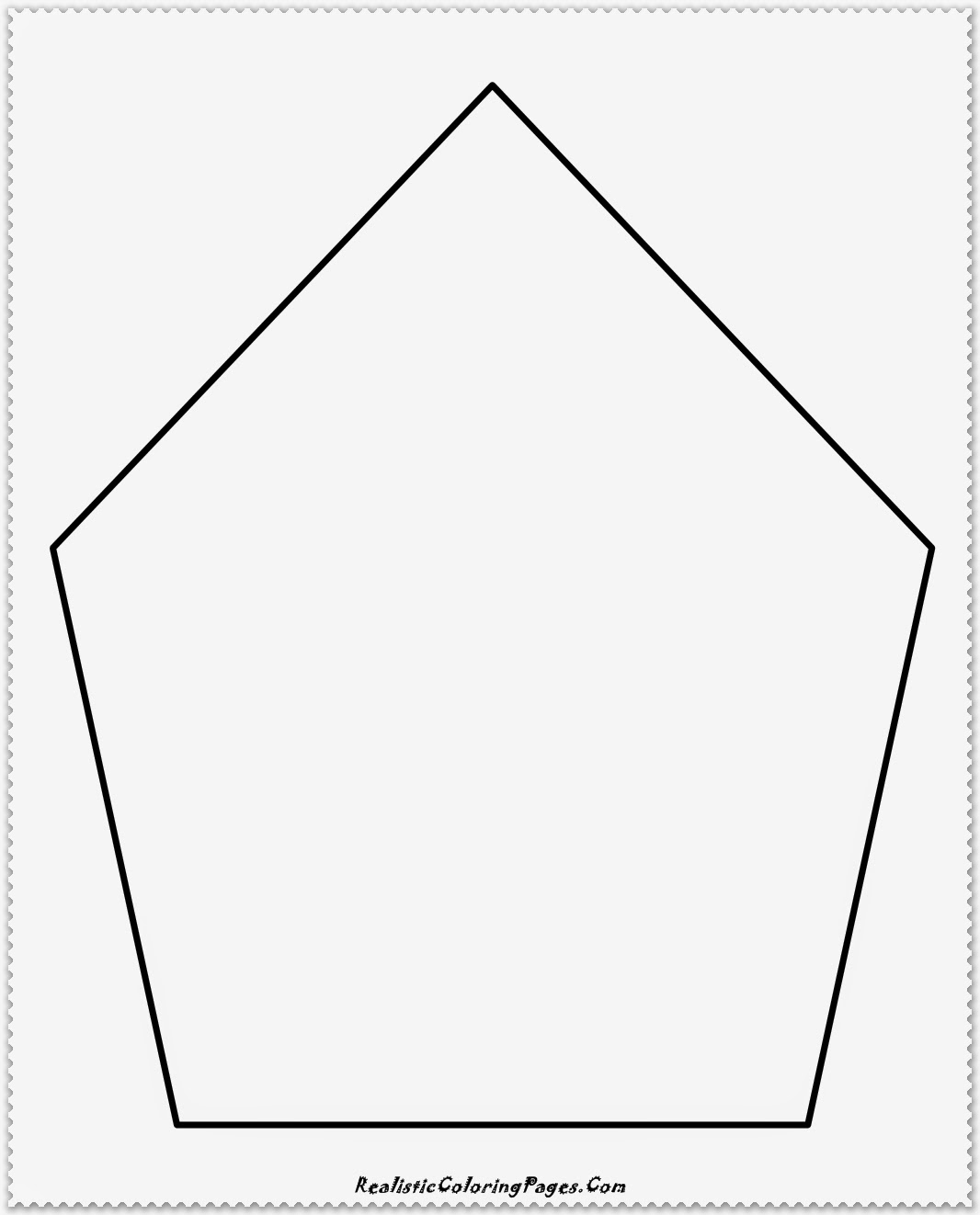The image showcases a clean, white piece of paper with roughly torn edges, giving it a somewhat serrated border. Dominating the center is a large, black-outlined shape resembling a pentagon, characterized by five straight edges with precise, sharp corners. The flat bottom edge of the pentagon tapers inward and ascends to a pointed top, strongly resembling a baseball home plate. At the bottom center of the paper, the text "realisticcoloringpages.com" is clearly printed in black. This simple yet detailed template is void of any other text or images, making it versatile for various activities such as tracing practice or creative drawing, potentially even being divided into segments for educational purposes like illustrating different seasons.